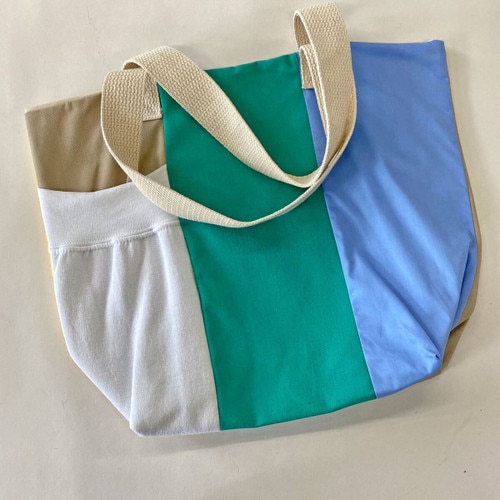This vertical rectangular photograph features a multicolored beach tote bag set against an off-white, slightly beige background. The bag is divided into four distinct vertical color sections. On the left side, there's a beige strip overlaid with a white mesh pocket, ideal for holding small items like a cell phone. The middle section features a green fabric stripe, while the right side showcases a light blue, almost powder blue, stripe. The tote is equipped with two off-white fabric straps with a visible woven texture; these straps are draped loosely over the front, predominantly covering the green and blue sections, with some of the strap attaching at the beige portion and draping over the white mesh pocket. Unique design features include the bag's slightly truncated bottom corners, enhancing its practicality for carrying items. The overall setting of the image, with its casual background and natural shadows, suggests it is not a professional product image.